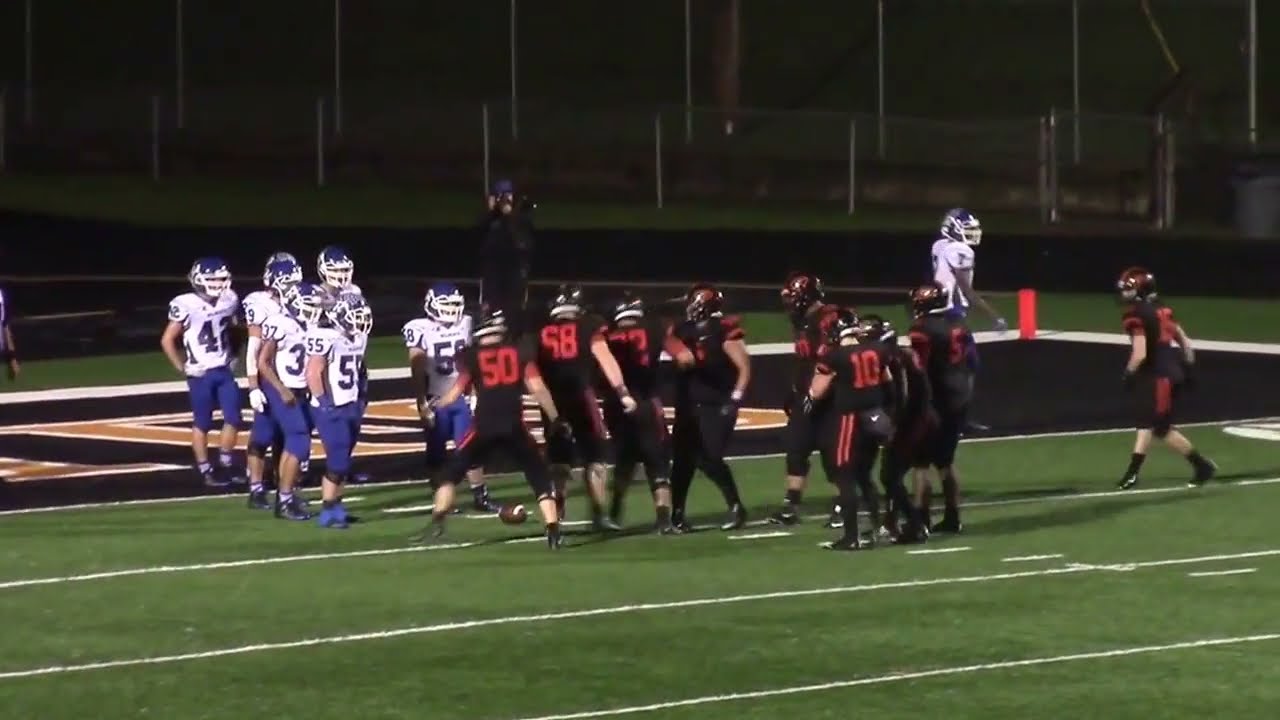This is a well-lit night-time outdoor color photograph capturing a high school American football game. The scene unfolds on a meticulously maintained green grass field with crisp white lines. The team with their backs to us wears black uniforms with vibrant red numbers; identifiable players include numbers 50, 58, 68, and 10. The opposing team, facing our direction, is dressed in white jerseys with blue numbers and blue pants; players 42, 58, 59, and 3 are visible.

The black team appears to be about five yards from the end zone, gearing up to snap the ball, while the white team lines up in defensive formation. The end zone behind the white team is emblazoned with gold letters on a black background. A photographer, positioned in the back corner of the end zone, is poised to capture the imminent play. Additionally, the background reveals a dark sky, indicative of night, and there's noticeable stadium lighting illuminating the field. A black strip, likely a track or pathway, runs parallel to a chain-link fence at the base of an ascending hill, framing the intense athletic moment.